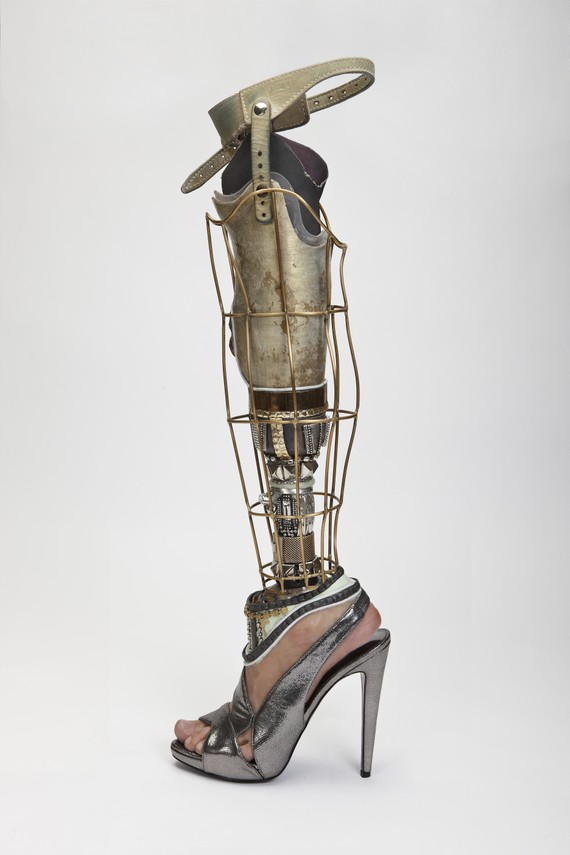This photograph features a detailed, old-timey prosthetic leg designed for a female, positioned upright on a dirty white backdrop. The lower portion showcases a realistic-looking, Caucasian-colored human foot, encased in a metallic gray, six-inch high-heeled shoe. Around the foot and extending up the calf is a complex wire framework interspersed with springs, resembling a steampunk or robotic aesthetic. This gives it some flexibility. From the ankle upwards, the prosthesis reveals its internal mechanics and lacks any covering, showing rust throughout the metal components, indicating significant use. The upper section of the prosthesis features a black attachment area that would sit around the amputated limb, secured by a gray strap. The overall design conjures images of a Victorian-era creation, blending art and functionality.